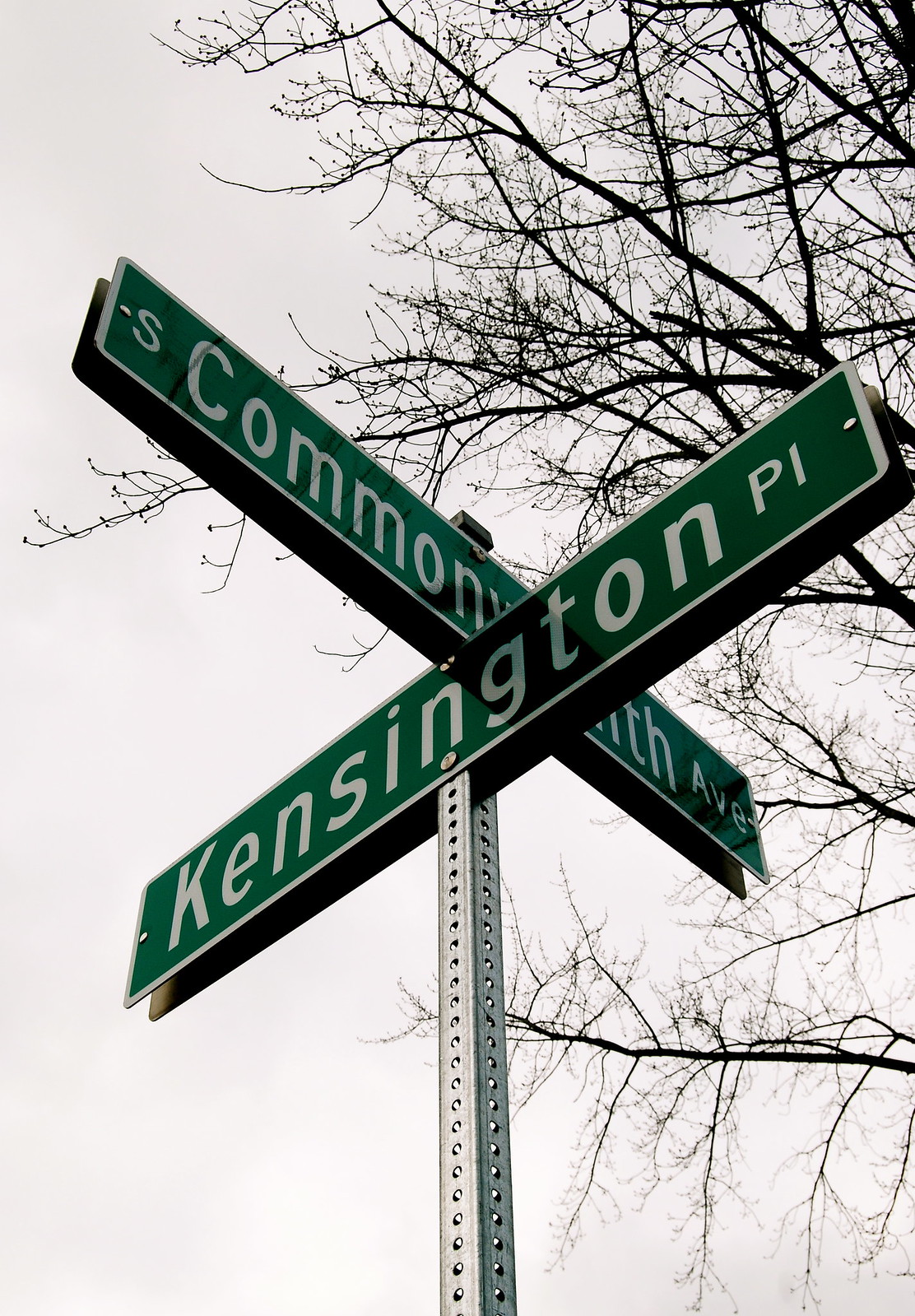The photograph captures a close-up view of an intersection street sign on a gray, silver pole. The pole supports two green, rectangular street signs arranged in an X shape at the top. One sign, pointing diagonally upward to the right, reads "Kensington Place" in white lettering against the green background. The other sign, crossing it horizontally at the top, reads "Commonwealth Avenue" in similar white letters on a green background. The daytime scene is characterized by a bright, white sky, likely obscured by a hazy cloud cover. Bare tree branches, indicating a winter season, span the background, devoid of leaves. The signs are affixed to the pole with visible silver screws, adding to the utilitarian aesthetic of the street corner.